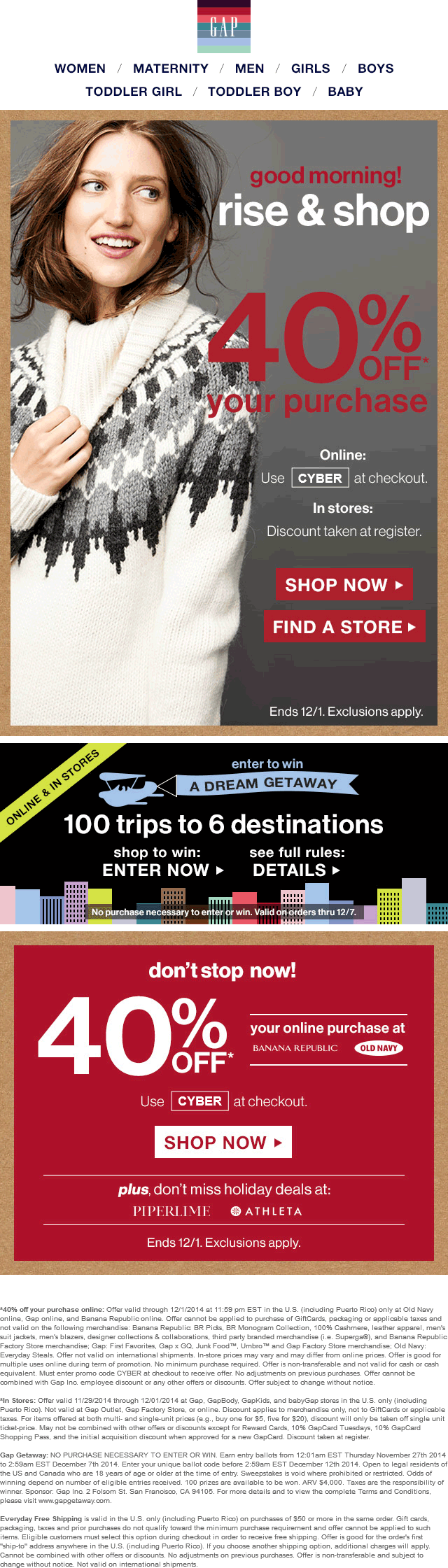The image showcases a vibrant advertisement for The Gap, prominently featuring the store's logo at the top in white letters against a multicolored background. Below the logo, product categories are listed: Women, Maternity, Men, Girls, Boys, Toddler Girl, Toddler Boy, Baby.

A central photograph captures a young, light-skinned woman with long, wavy brown hair, smiling and looking to the right. She is dressed in a collared sweater with a black, white, and gray pattern. Text superimposed on this section reads: "Good Morning. Rise and shop. 40% off your purchase. Online use 'Cyber' at checkout. In stores, discount taken at register. Shop now. Find a store. Ends 12-1. Exclusions apply."

Beneath this, a black banner depicts a cartoon skyline with an airplane towing a banner that announces: "Enter to win a dream getaway. Online and in stores. 100 trips to 6 destinations. Shop to win. See full rules, details. No purchase necessary to enter or win. Valid on orders through 12-7."

Further down, a red rectangle highlights another promotion: "Don't stop now. 40% off your online purchase at Banana Republic, Old Navy. Use 'Cyber' at checkout. Plus don't miss holiday deals at Piper Lime, Athleta. Ends 12-1. Exclusions apply."

At the very bottom of the image, there is fine print that is too small to read legibly.